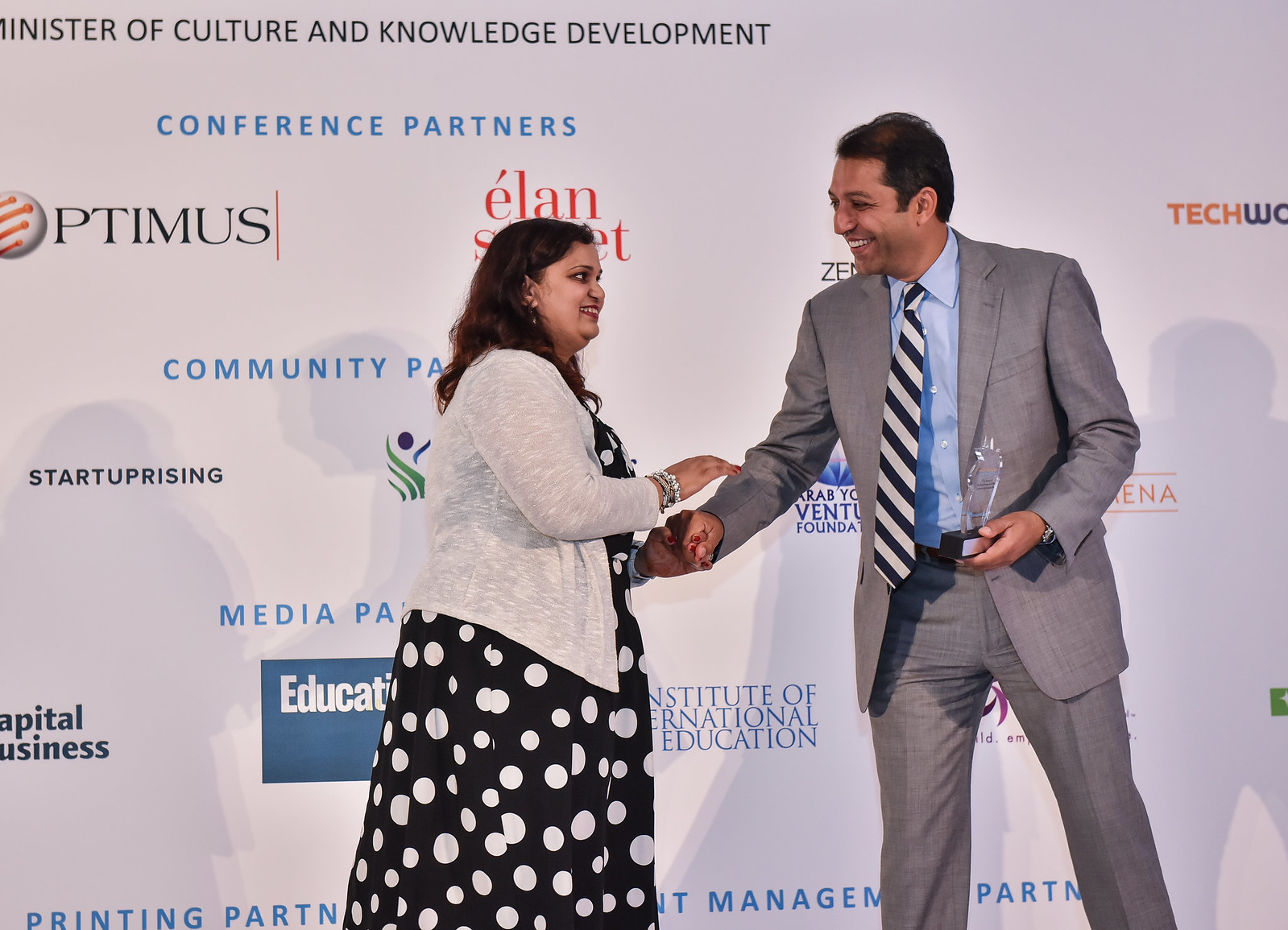In this photograph, a man and a woman, both appearing to be of Indian descent, are pictured shaking hands and smiling at each other. The woman, positioned on the left, has long, dark hair and is dressed in a black, long-sleeved dress adorned with white polka dots, complemented by a white cardigan sweater. She is smiling warmly, showing her top teeth, and has a couple of bracelets around her right wrist. The man, standing to her right and a head taller, has short black hair and is attired in a light gray suit, a blue button-down shirt, and a black-and-white striped tie. He is holding a clear, glass award plaque in his left hand and is also smiling, with his eyes partially closed. In the background, a white wall displays various sponsor logos such as Optimus, Startup Rising, and Capital Business. At the top of the wall, bold black text reads, "Minister of Culture and Knowledge Development, Conference Partners." This image captures the joyful moment of an awards presentation.